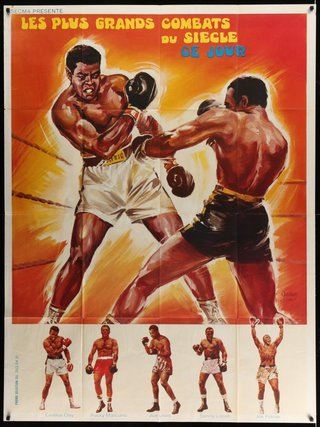The illustration showcases a dynamic boxing scene set against a red background, bordered by a white frame with black edges and pinned corners. At the top, French text hints at an epic combat event. The main focus is on two boxers in a ring, where the fighter in black trunks delivers a forceful left jab to the midsection of his opponent, who is clad in white trunks, guarding himself with gritted teeth and a downward gaze. Both boxers sport gold belts, signifying their champion status. Below the primary image, five other boxers appear, with some raising their hands in victory and others presenting their fists, possibly celebrating or preparing for their own bouts. The illustration is rendered in a cartoony, impressionist style, creating a vibrant and energetic atmosphere reminiscent of classic boxing advertisements.